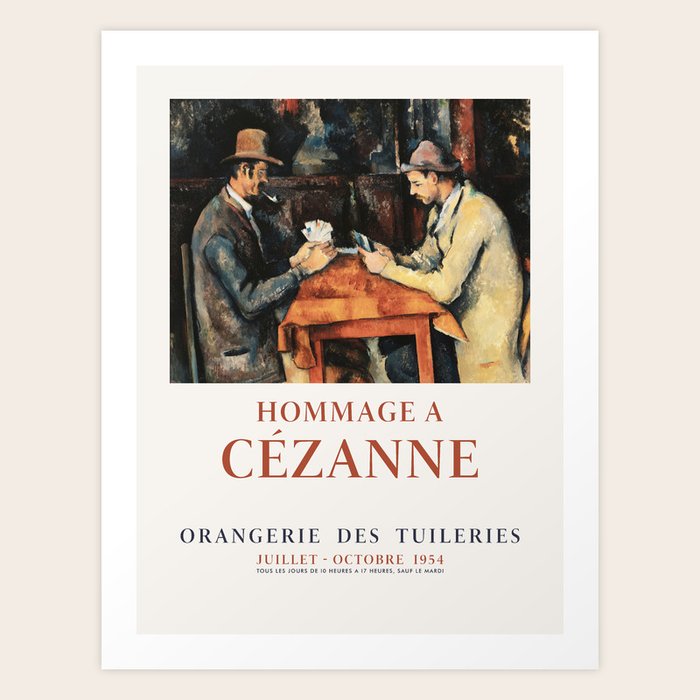The image depicts a digital representation of a poster, set against a grey background bordered in white and green. The central focus is a painting of two Caucasian men sitting at a small, brown table with a brown tablecloth, engaged in a game of cards. Both men, one wearing a dark-colored suit with a brown hat and the other donned in a tan trench coat with a brown hat, are playing cards. The man in the dark suit looks wealthier compared to the one in the trench coat. One of the men also holds a pipe.

Above the image is an artistic representation of a painting, and below it, text details are displayed in various colors and fonts. The red, all-caps text reads "HOMAGE A CÉZANNE," indicating the painting is a tribute to the famous French artist Paul Cézanne. Beneath that, in black, all-caps letters, it states "Orangerie des Tuileries," followed by the exhibition dates "July-October 1954," which is also written in French.